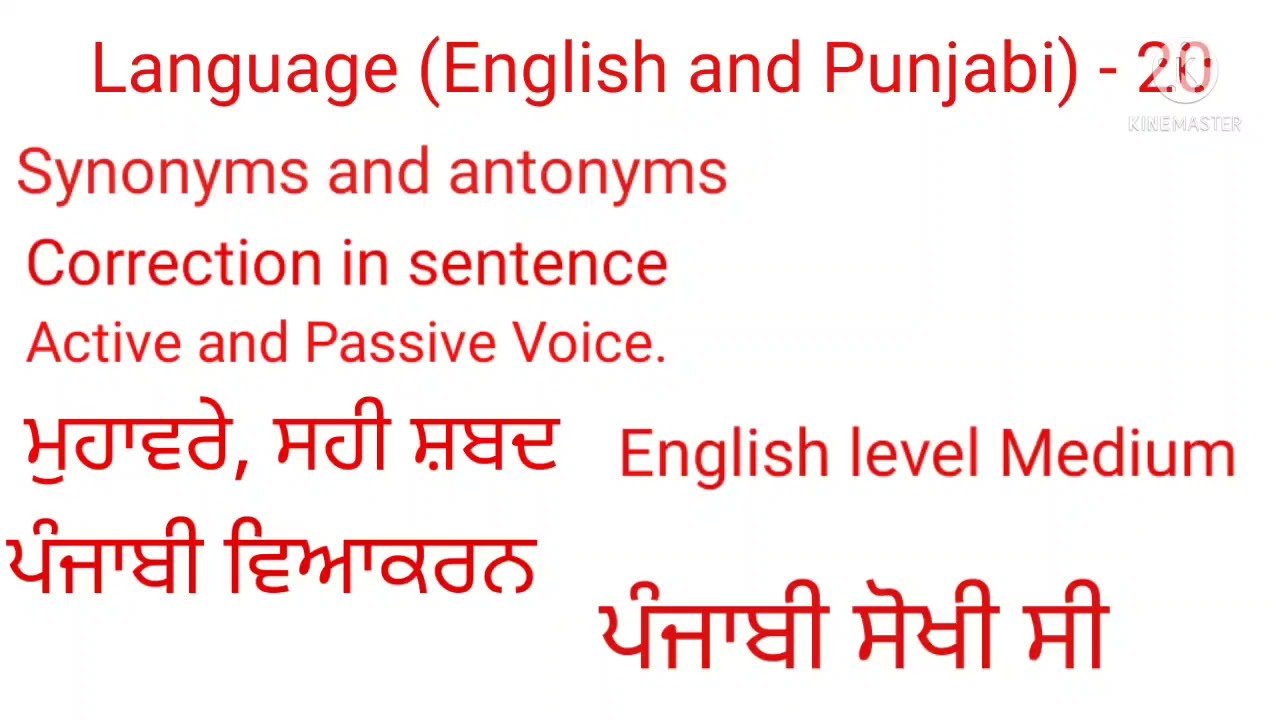The image features a plain white background with striking red text, bordered by no additional imagery. At the top center, the text reads "Language (English and P-U-N-J-A-B-I) - 20." Directly beneath this, aligned to the left, are the segments "synonyms and antonyms," "correction in sentence," and "active and passive voice." Following these lines are two rows of foreign language text on the left. To the right of this foreign text, the words "English level medium" are prominently displayed. Additionally, in the upper right corner, there is a small circular logo featuring the letter "K" encircled, accompanied by the word "KineMaster" underneath. Together, there are six or seven lines of text in total, with the entire text content displayed in red.